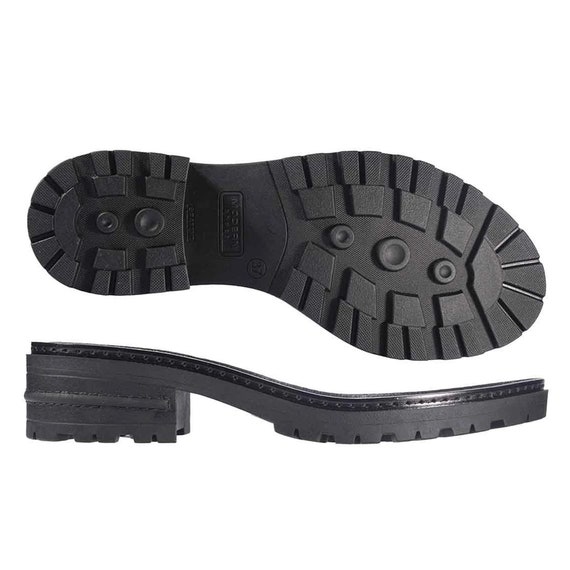This image features the sole of a black shoe presented in two different views. The top part of the photograph shows a direct bottom view of the right shoe's sole, emphasizing its complex tread pattern. The sole is predominantly black and made of rubber, showcasing excellent traction with intricate, circular, and uneven treads along the perimeter and three rubber dots at the front, plus two at the heel. The lower part of the image provides a side view of the sole, highlighting the shoe's one-inch high heel and the areas designed for stitching. The detailed tread pattern and durable material suggest significant emphasis on functionality and grip. The presentation of these views, one from the bottom and one from the side, might be targeted for a product detail page on a website selling footwear, highlighting the shoe's tread and construction quality.